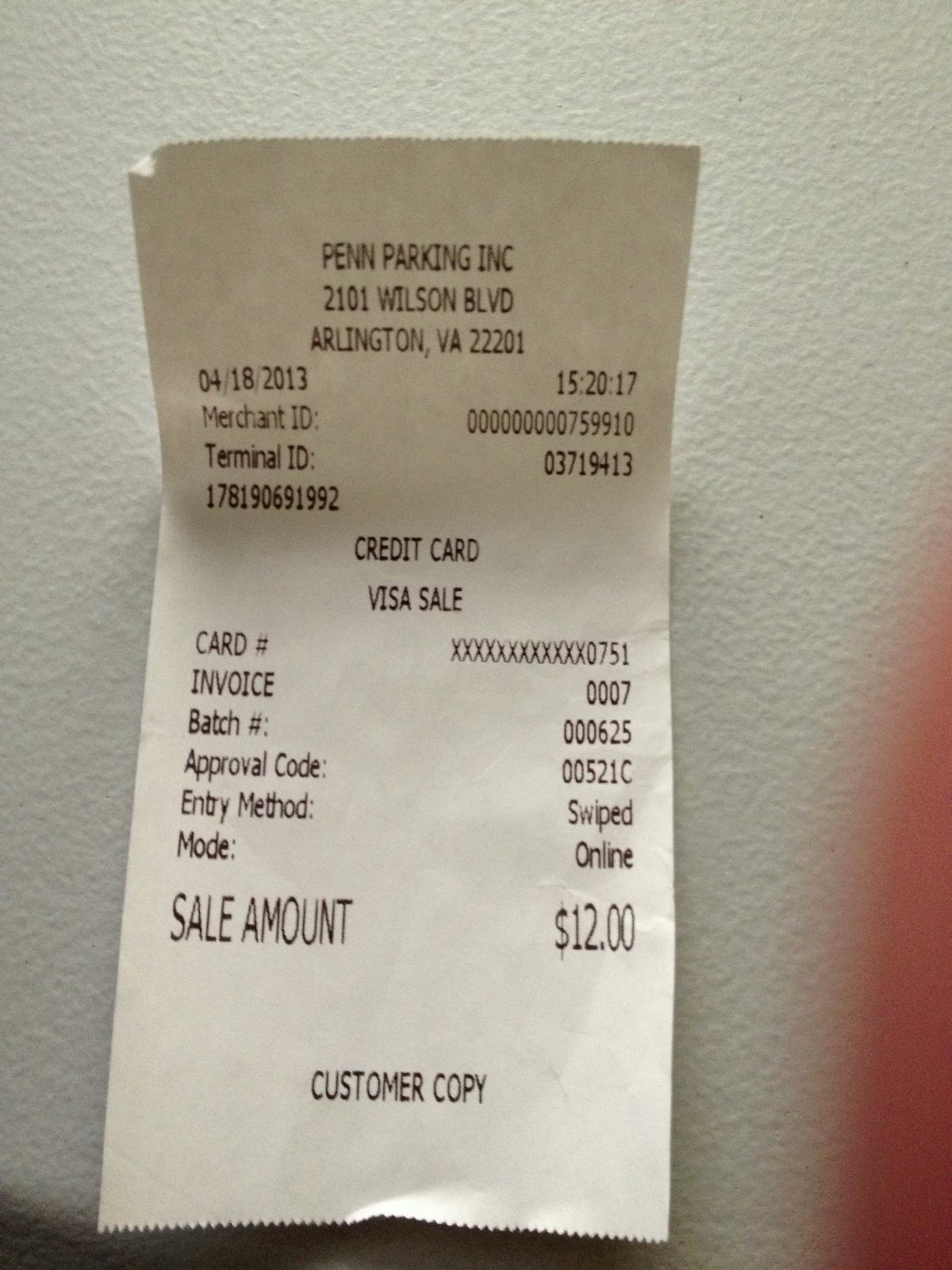This photograph captures a close-up of a receipt laid on a textured white surface. On the right edge, a blurred tip of a thumb or finger is visible, indicating that someone is holding the receipt. The receipt has a distinct fold about a third of the way from the top, causing the upper portion to angle slightly upwards. At the top, the text is centered and printed in black capital letters, reading "PENN PARKING INC." Below this, the address "2101 Wilson Boulevard, Arlington VA 22201” is detailed. Further down, the receipt includes specific transaction details such as the date, time, merchant ID, and terminal ID. A large number is listed under the terminal ID. Following this, the words "CREDIT CARD" and "VISA SALE" are centered on the receipt. The credit card number is partially obscured, with the first 12 digits replaced by X's. Below this are fields for the invoice number, batch number, approval code, entry method, and mode issued. At the bottom, the sale amount of $12 is highlighted, with "CUSTOMER COPY" printed in centered capital letters beneath it.